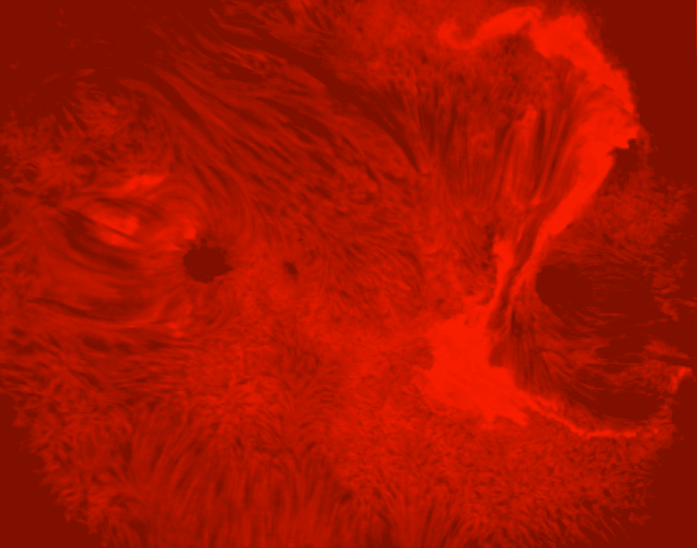This large, square, borderless image features an abstract visual reminiscent of waves or fluid motion. Dominated by varying shades of red, the image transitions from darker, maroon-like tones at the corners to lighter reds and reddish oranges toward the center. The texture in the image is dynamic, resembling feathery waves or possibly fluid mixtures, such as lava or sunspots. Notably, there is a small, circular hole marked by dark reddish-orange coloration on the middle left side, adding a point of interest. On the right side, a distinctive C-shaped wave-like formation can be seen, characterized by a thicker border at the top resembling the tip of a wave, which thins out towards the bottom. The abstract nature of the image evokes multiple interpretations, ranging from a microscopic view of a porous surface to an artistic rendering of turbulent, colorful waves.